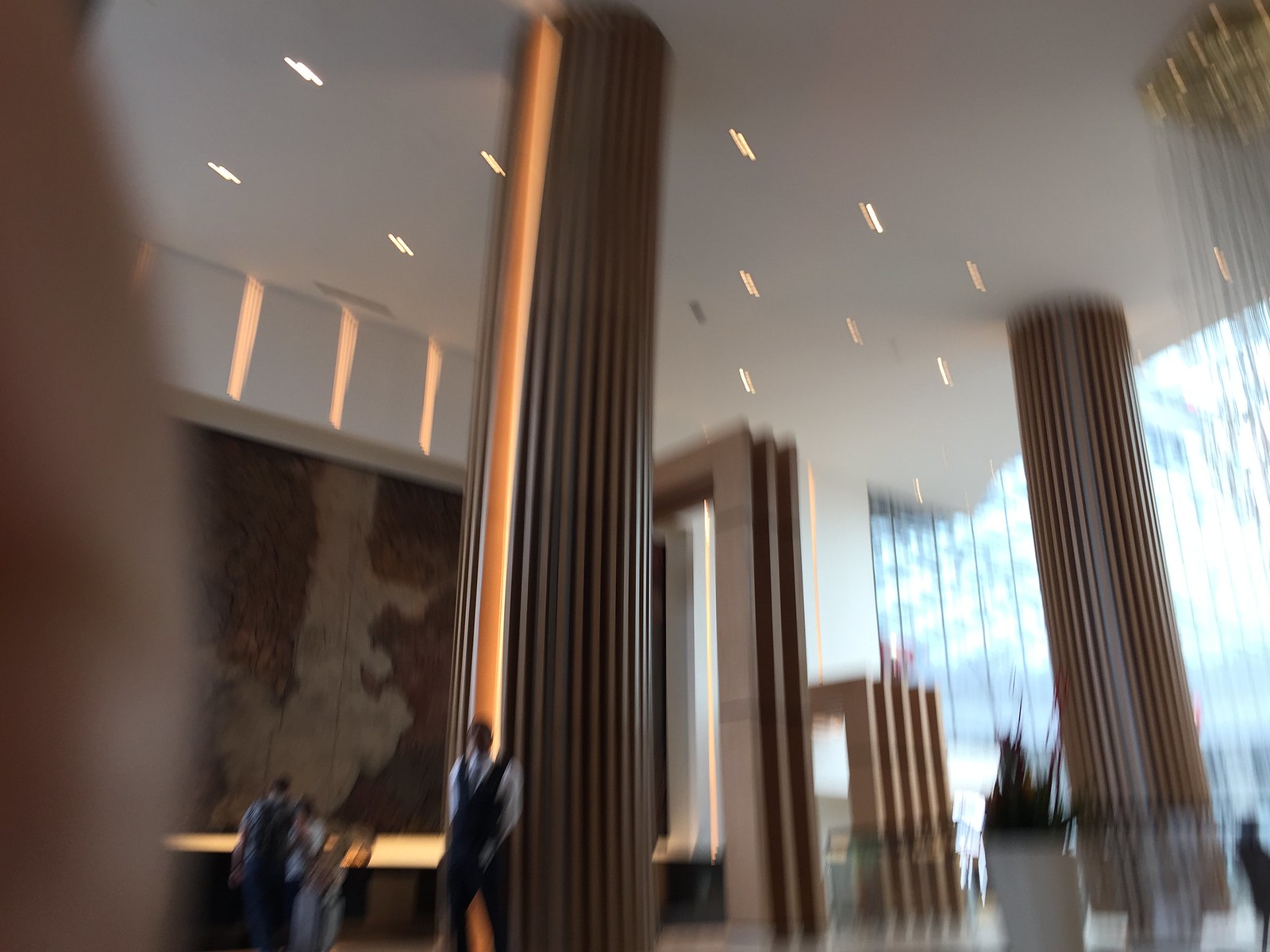The image depicts a large, blurry interior of a grand building with very high ceilings adorned with hanging lights and chandeliers. Notably, a long, cascading chandelier is situated to the right, casting intricate shadows on the ceiling. The room features tall, striped brown pillars extending from the floor to the ceiling. A gentleman, dressed in a white long-sleeved button-up shirt with a tie, a black vest, and black dress pants, stands in front of one of these pillars. To the left of the gentleman, a couple appears engrossed in a lit display case, nearby which an antique-looking map is mounted on the wall below upward-facing lights. The floor is shiny, reflecting parts of the structure, and greenery is visible within the scene. On the left edge of the photo, there's an obstruction, likely someone's hand or finger. Large glass windows are also visible to the right. The image appears to have been taken hurriedly or while in motion, contributing to its blurred quality.